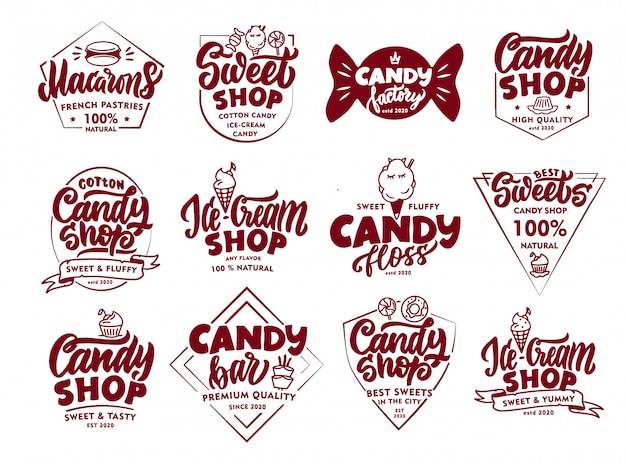The image showcases 12 distinctive company logos, all themed around sweets and confections, arranged in a horizontal rectangle with a white background. The logos are organized into three rows and four columns, each intricately designed in variations of dark maroony red. The top row features a variety of candy and shop themes: the first logo depicts the front of a building with a hamburger image and "macarons, 100% natural" written on it. To its right, another logo, rounded at the bottom and square at the top, includes a giraffe holding candy and reads "Sweet Shop, Cotton Candy, Ice Cream and Candy." Next is a wrapped piece of candy labeled "Candy Factory." The rightmost logo in the top row resembles a house and says "Candy Shop, High Quality."

Moving to the second and third rows, each logo continues with the confectionery theme, depicting items like ice cream and cotton candy, each featuring unique branding such as "Cotton Candy Shop, Sweet and Fluffy," "Ice Cream Shop, 100% Natural," "Candy Floss, Sweet and Fluffy," "Sweets Candy Shop, 100% Natural," “Candy Shop, Sweet and Tasty," "Candy Bar, Premium Quality," "Candy Shop, Best Sweets," and "Ice Cream Shop, Sweet and Yummy." All text is prominently displayed in bright red against the white background.